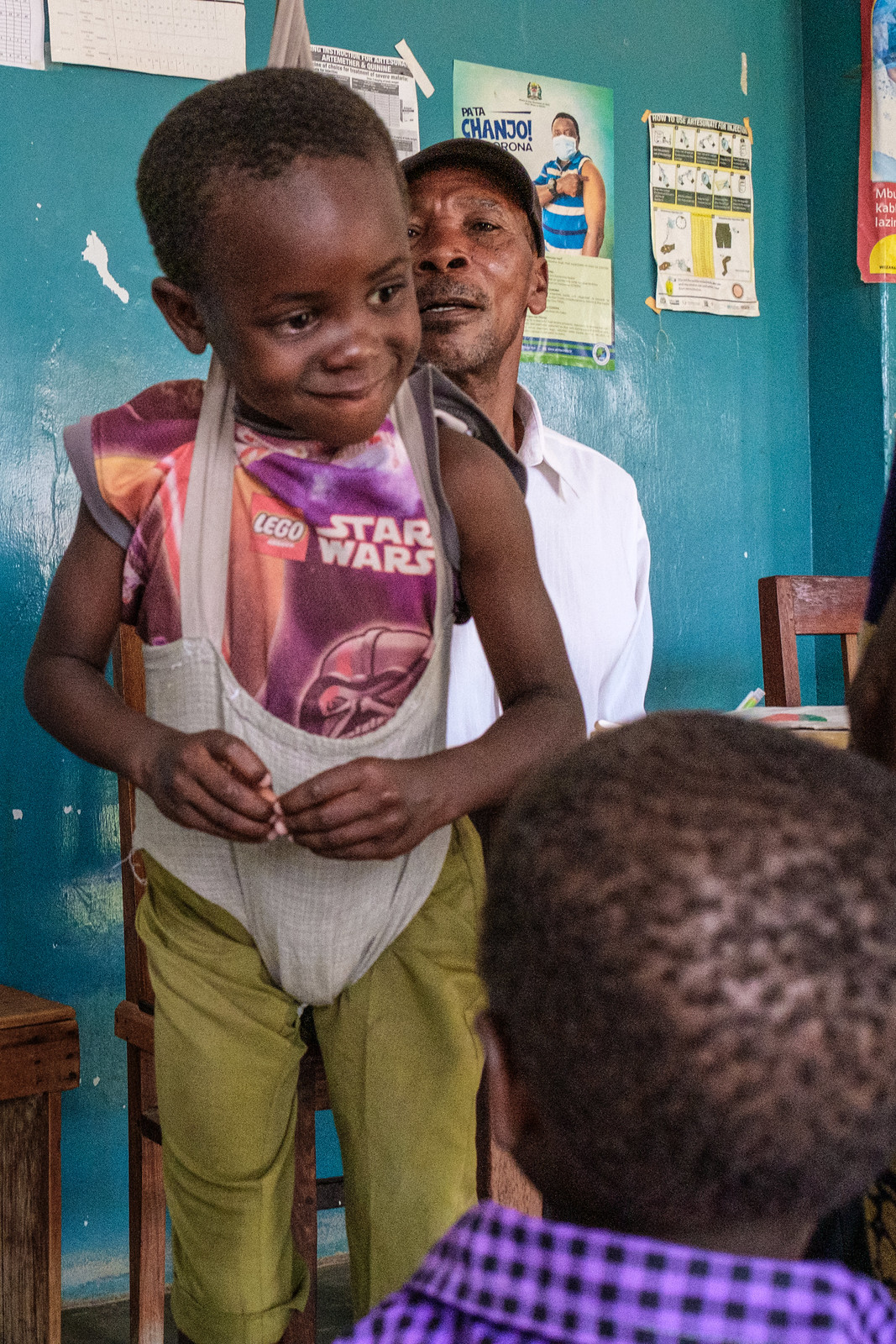In this evocative photograph, we find ourselves in a possibly rundown classroom typical of a developing country. The background features blue walls with visible chips and a few taped-on signs, one of which displays an image of a man in a mask pointing to his arm, likely promoting vaccination.

At the forefront, a young African boy, wearing a green pair of pants and a distinctive Lego Star Wars T-shirt, stands facing the camera with a bemused expression as if he just shared a joke. He is clad in an unusual outfit that appears to be some sort of onesie or bib-like garment, with what seems like underwear awkwardly stretched up behind his neck, creating a peculiar impression of a wedgie. 

Behind him sits an older African man, probably in his 40s, distinguished by his graying hair, baseball cap, and white button-down shirt, suggesting he might be the teacher. In the lower corner of the frame, the back of another young boy's head is visible; he is wearing a black and blue checkered collared shirt. The entire scene is tightly cropped, focusing on these key figures and the wear and tear of their surroundings.